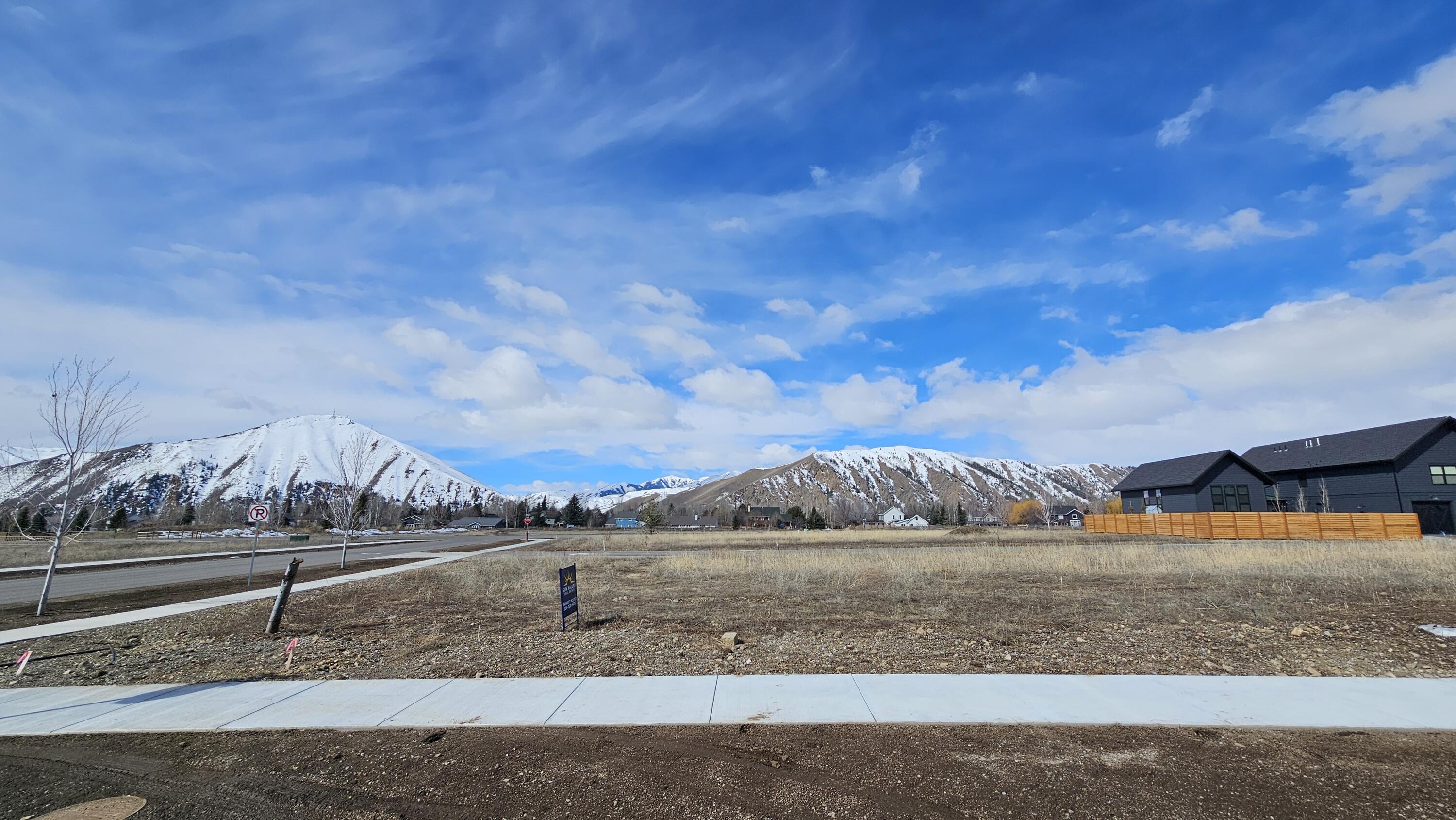The photo captures a scenic daytime landscape featuring a bright blue sky scattered with puffy white clouds. In the background, snow-capped mountain ranges rise dramatically, providing a striking contrast to the mid-ground. To the right of the image stands a black building, likely a barn, enclosed by a brown wooden fence. Adjacent to this structure, there's a stretch of vacant land, primarily filled with dirt and sprinkled with patches of grass and rocks. Cutting through the barren lot is a wide white sidewalk running horizontally across the lower third of the frame, intersecting a road on the far left, which winds its way toward the mountains. A sign, possibly indicating no parking, can be seen along the sidewalk. Further forward from the mountains, a row of smaller, darker houses lines the scenery, adding depth to the residential feel of the image.